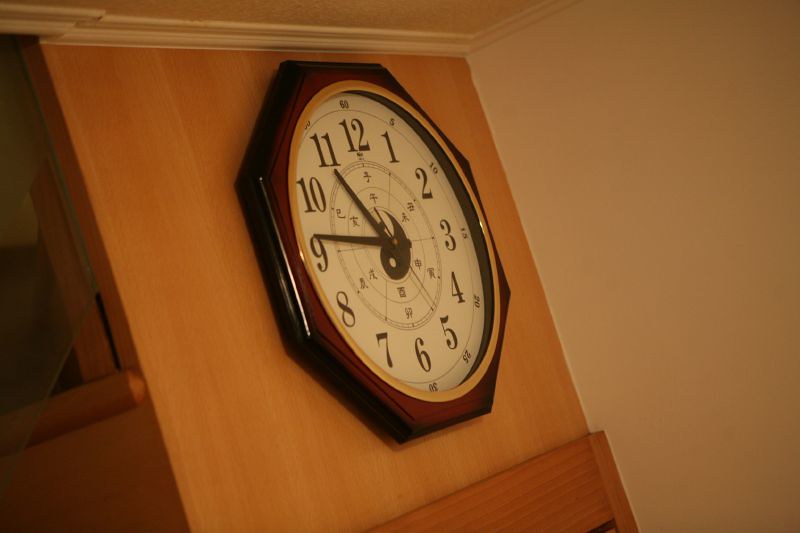This photograph captures a wall clock adorned with a white face featuring a central illustration depicting a moon and a sun. The black hour, minute, and second hands emerge from this celestial design, precisely indicating the time against bold black numerals ranging from 1 to 12. Encircling the clock face is a refined gold casing, further accentuated by an outer border crafted from dark cherry wood, shaped into a soft-edged octagon. The entire piece is elegantly mounted on a light oak-colored wooden panel, possibly part of a larger furniture piece such as a shelf.